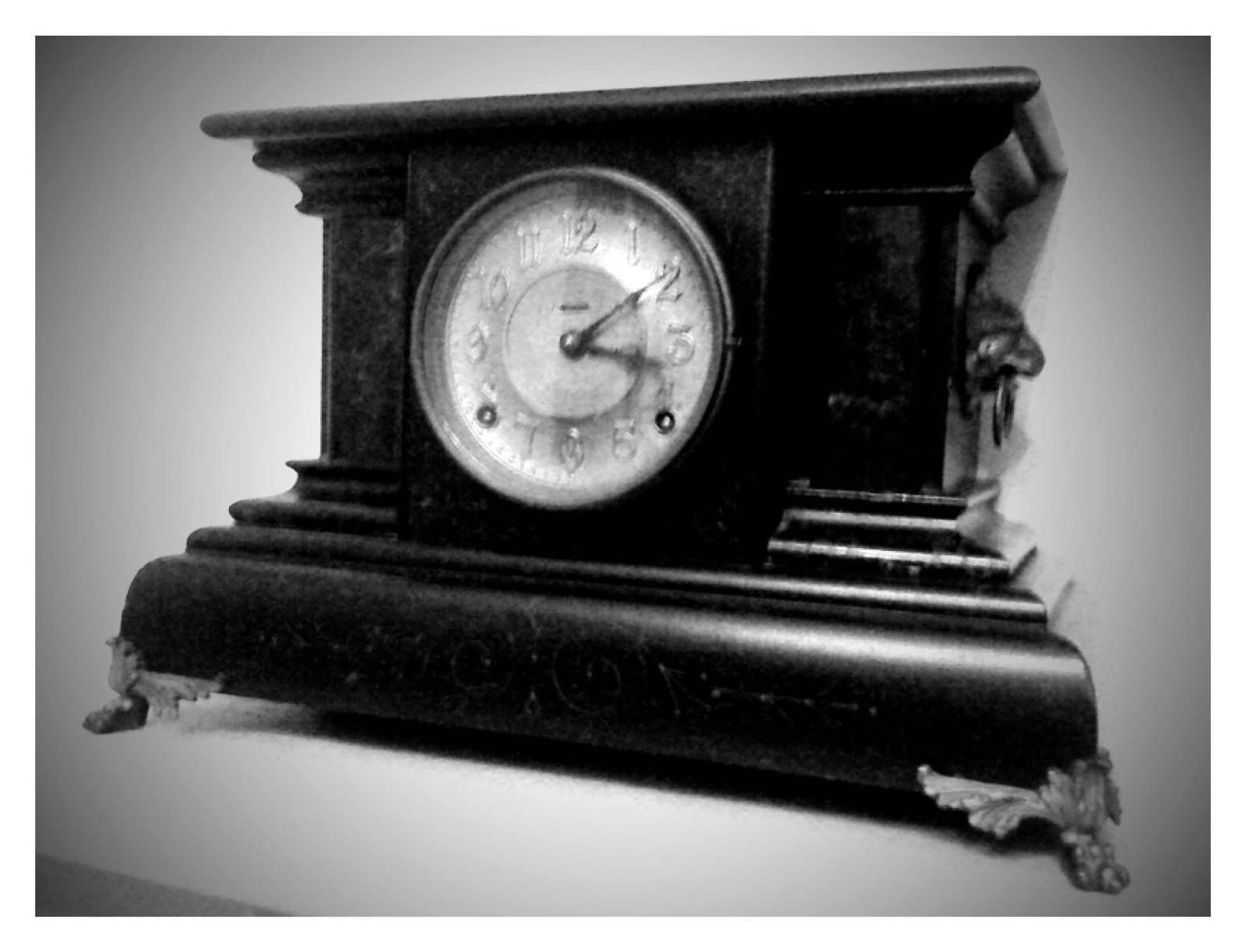This black and white photograph features an elegant, antique clock, possibly crafted from a single piece of dark wood—likely dark brown or black. The clock, positioned against a background that appears grayish or white, showcases exquisite craftsmanship. It is adorned with gold accents, including ornate feet and fittings around the white clock face. The clock's hands indicate the time as 3:10, though whether it is morning or afternoon is unclear. The numerals and finer details may also be gold, though this is uncertain due to the monochromatic nature of the image. The photo itself could be either genuinely old or designed with a black and white filter to evoke a vintage feel.